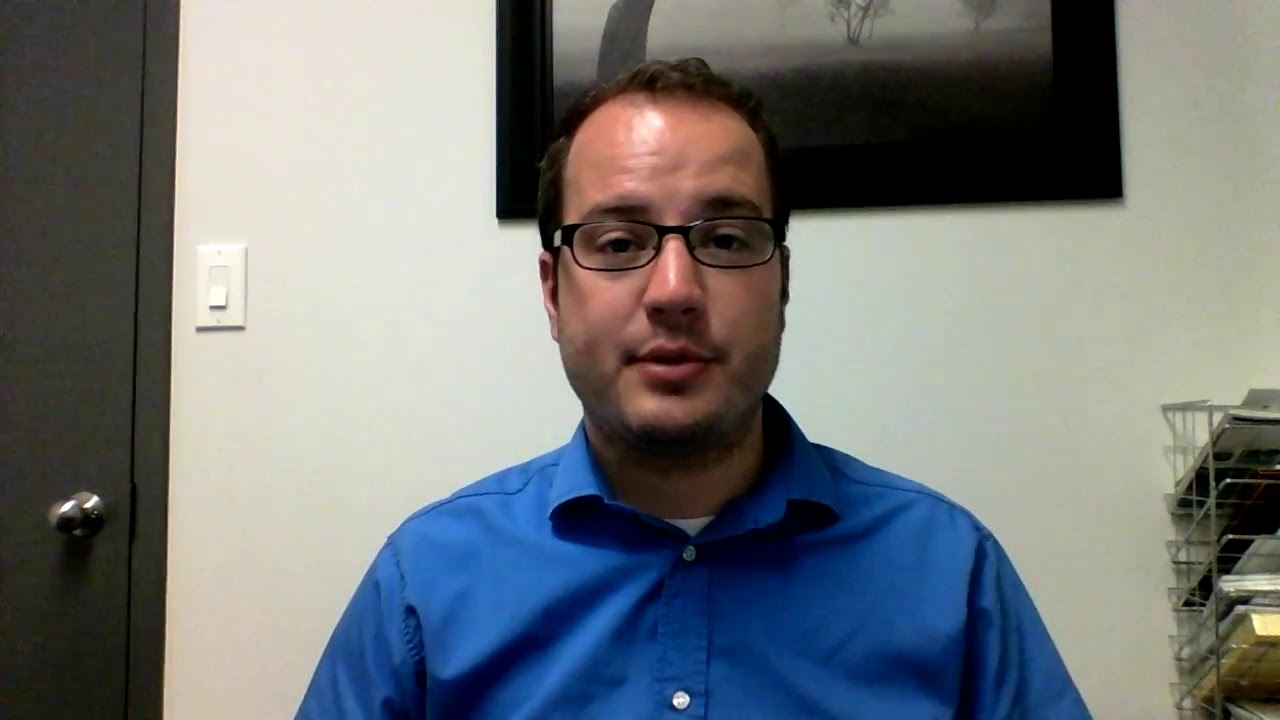A white male with short, receding black hair, thin black-rimmed rectangular glasses, and slightly shiny skin sits in a room, staring directly at the camera with his mouth partially open as if speaking. He wears a blue, buttoned-up collared shirt with white buttons, revealing a white shirt underneath. Behind him, a black-framed photograph depicting a foggy forest with thin tree branches and a dark brown floor hangs on a white wall. To the left, a closed black door with a silver knob is positioned next to a white light switch. On the right, a five-tier metal filing tray holding an assortment of books and papers can be seen.